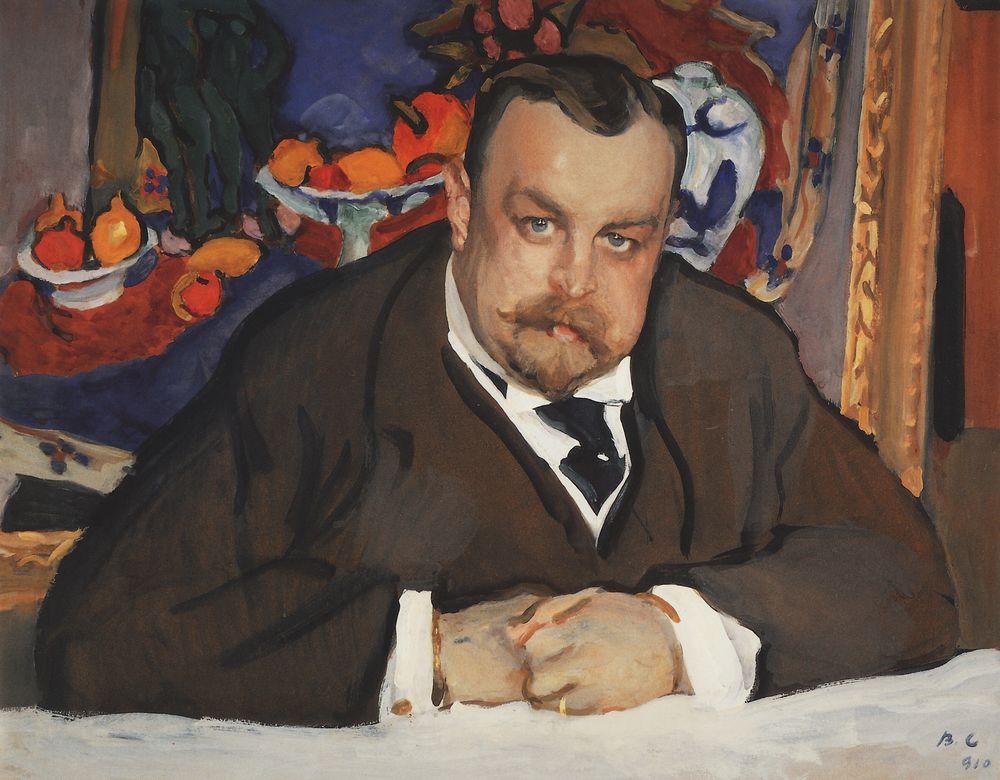The image depicts a detailed and expressive painting of a stout gentleman reminiscent of former President Taft, sitting at a white table. He presents with a composed demeanor, with his hands folded and resting on the table's surface, possibly indicating a sense of contemplation or reflection. The man has short, slicked-back brown hair, accompanied by a receding hairline forming a widow's peak, and features a brown mustache and goatee. His kindly blue eyes gaze slightly right, beneath prominent, arching eyebrows, suggesting a thoughtful expression.

The gentleman is dressed in a vintage-style brown suit with a white collared shirt and a black tie neatly tucked into his suit, adding to his dignified appearance. Noticeable accessories include a gold ring on his left pinky finger, a gold cufflink, and a gold watch on his right wrist, further enhancing his distinguished look.

The background showcases an elaborate and vividly colored painting framed in an ornate wooden frame. This secondary painting within the painting features an array of brightly colored fruits, including lemons, apples, and oranges, displayed in various bowls. Complementing these bowls is a white and blue vase, adding to the still life’s richness, set against a vivid blue backdrop with hints of green from trees. Intriguingly, the bottom right-hand corner of this background painting bears the artist's initials "B C" alongside an ambiguous notation that seems to be a number, possibly "910" or a symbol resembling "$10."

This composition not only highlights the central figure’s imposing presence but also showcases the meticulous detail and vibrant colors of the artwork behind him, creating a captivating double-layered imagery that speaks of both the subject and the artist's prowess.